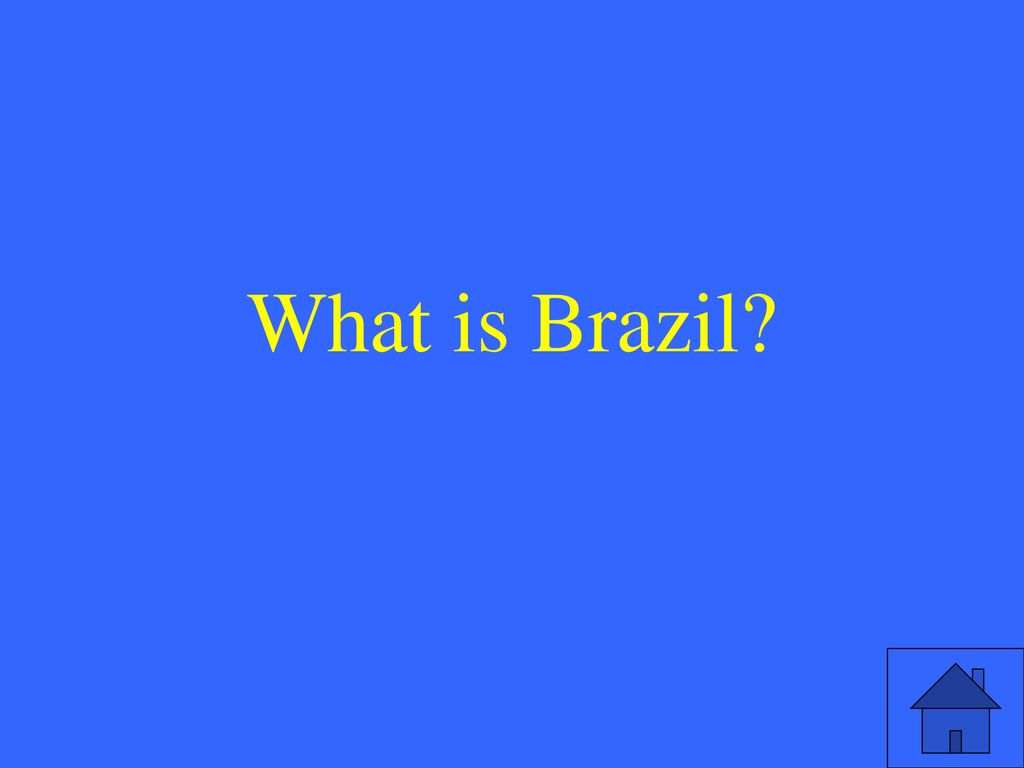The image features a solid blue background encompassing the entire frame. In the bottom right corner, there is a small square outlined with a thin black line. Within this square, a simplistic, 2D house is drawn. The house consists of a triangular roof shaded in a dark color, and its walls are represented by a square shaded in light gray. The door, a small rectangle, and the chimney on the top right of the roof are both shaded the same color as the roof. This drawing is rendered with crisp, straight lines forming distinct angles and shapes including triangles, squares, and rectangles.

Centrally positioned in the image, there is a text in bright yellow that poses a question: "What is Brazil?" The text stands out against the blue background, with a question mark at the end. The entire design focuses on the clear contrast between the blue background and the elements drawn and written in other colors.